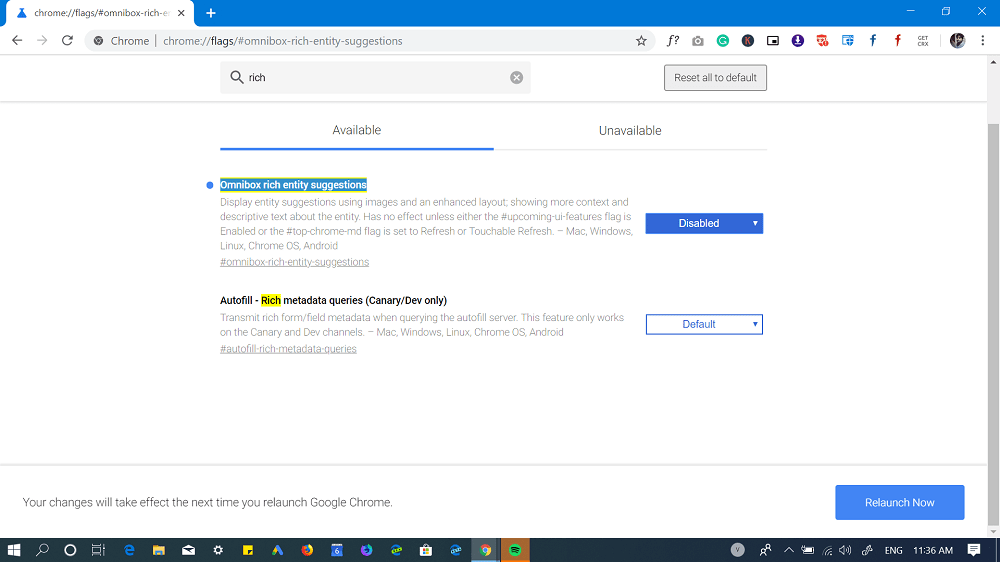The image is a detailed screenshot of the Chrome browser's experimental features page, accessible via "chrome://flags". The main page features a minimalist design with a white background and ample empty space. The browser tab is singular and shows "chrome://flags" in the address bar. The page header is blue, and the browser toolbar includes several icons to the right of the search bar, alongside an arrow and a refresh button to the left.

Dominating the central part of the screen is a search bar with a magnifying glass icon, displaying the term "Rich" in both normal and highlighted forms with a background yellow color on the keyword "Rich". A "Reset All to Default" button is situated to the right of the search bar. Below, the page is divided into two sections: "Available" and "Unavailable," with the "Available" category underscored in blue.

Within the "Available" section, the first result listed is "Omnibox Rich Entity Suggestions," accompanied by a paragraph of light gray explanatory text and a blue disabled button to the right. Directly under this entry is the "Autofill Rich Metadata Queries, Canary/DEV Only" option. This entry also has explanatory text in light gray and an unselected default button beside it.

At the bottom left of the screen, a message states, "Your changes will take effect the next time you relaunch Google Chrome." A prominent blue "Relaunch Now" button is positioned on the right side. The image also includes a vertical scrollbar on the far right edge, with a black footer bar hosting several icons extending across the screen both to the left and right sides.